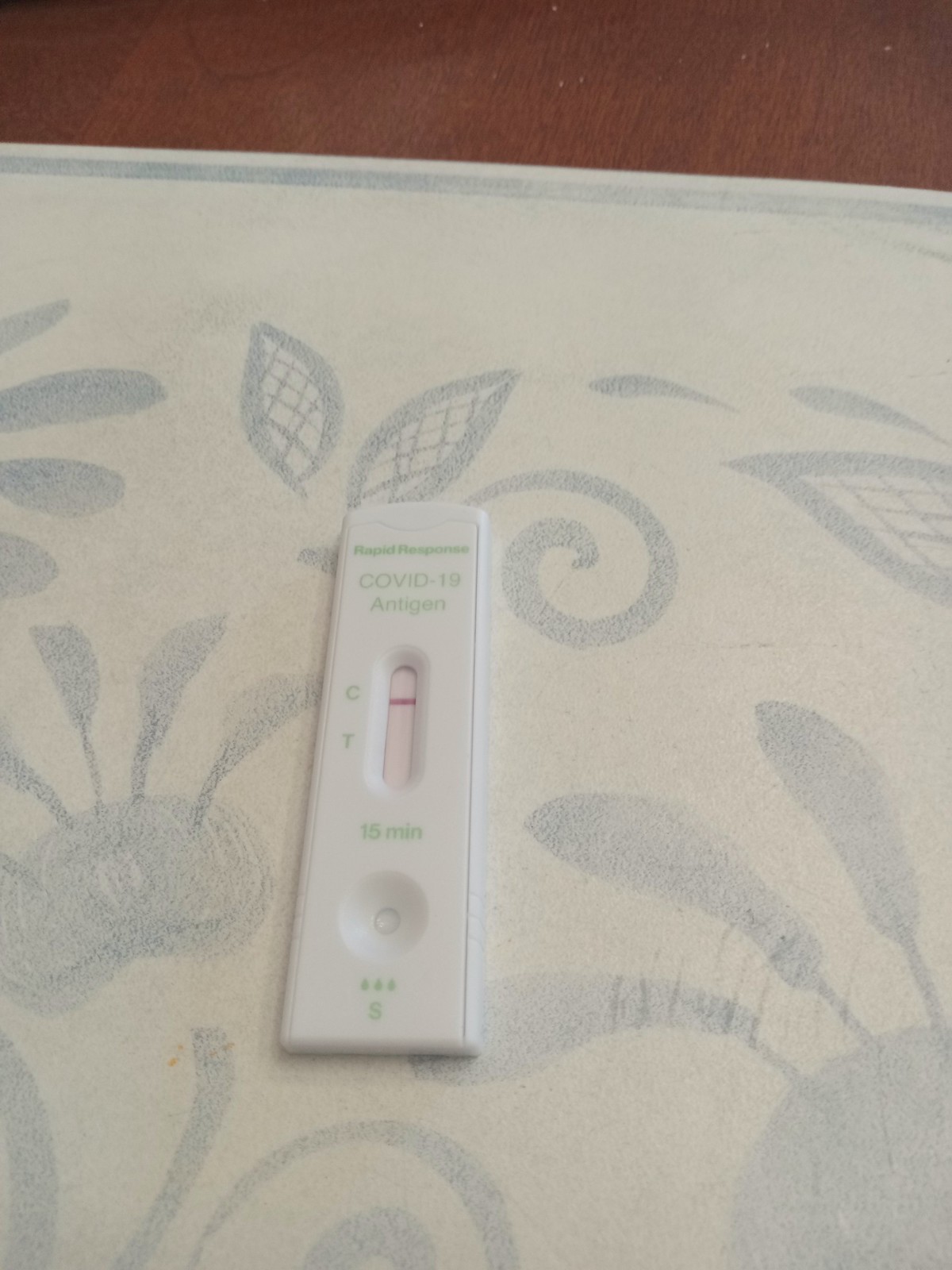The image features a gradient brown background that thickens towards the right and thins towards the left. Overlaying this background is a distinctly off-white object adorned with intricate gray-blue patterns, including swirls and leaf-like shapes that are criss-crossed inside. Additional circle patterns are visible, with one full circle on the lower right-hand side and part of a circle on the lower left-hand side. The off-white area subtly transitions to a pinkish hue in the center.

Prominently displayed on this backdrop is a white rectangular object. The text "rapid response" is written in green at the top, followed by "COVID-19" and "antigen" in the same green font beneath it. Positioned within this white object is an oval-shaped window with a light pink hue, featuring a dark pink line inside the window. To the left of the oval window are the letters "C" and "T". Below this section, it reads "15 minutes," accompanied by a circular icon with a smaller circle inside it and additional green lettering that is too small to decipher, followed by the number "5".